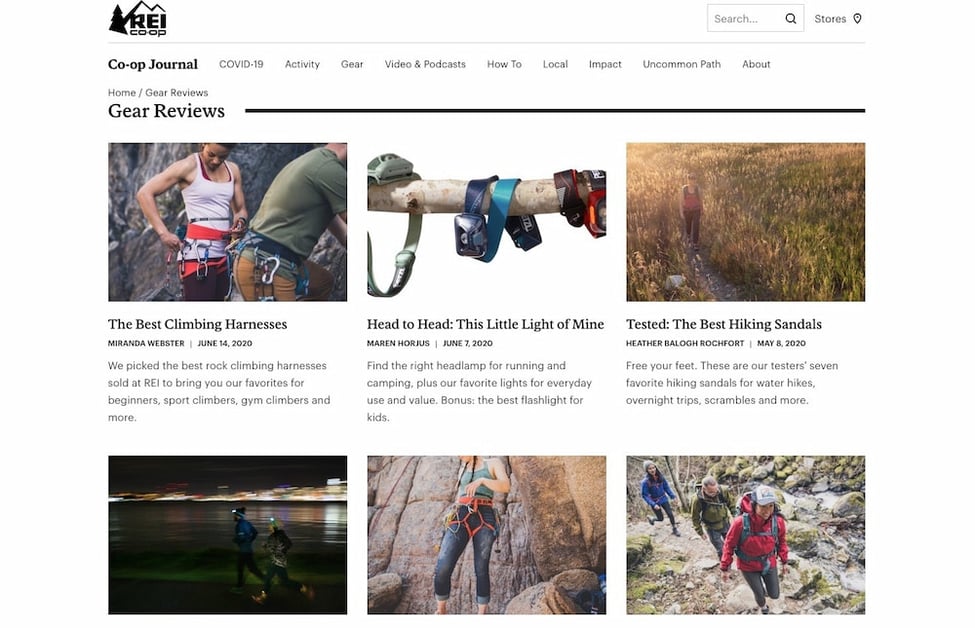This is a detailed screenshot from the REI Co-op website. At the top of the page, the REI Co-op logo is prominently displayed, featuring a line drawing of a mountain range and a pine tree juxtaposed with the company's name. The navigation bar includes categories like Search, Stores, Co-op Journal, COVID-19, Activity, Gear, Video and Podcasts, How-to, Local, Impact, Uncommon Path, About, Home, and Gear Reviews.

The main section of the page highlights articles with images. The first feature displays a photo of two individuals gearing up for mountain climbing. The caption reads, "The Best Climbing Harnesses," written by Miranda Webster, June 14, 2020. The description indicates a selection of rock climbing harnesses available at REI, recommended for beginners, sport climbers, gym climbers, and more.

Below this, there is an image of various headlamp straps draped over a branch. The caption for this image, titled "Head-to-Head: This Little Light of Mine," is authored by Maren Horges, June 7, 2020. This section advises on choosing the right headlamp for running and camping, highlighting favorite lights for everyday use and value, and includes recommendations for the best flashlight for kids.

The next image features an individual traversing a grassy field. The caption states, "Tested: The Best Hiking Sandals," written by Heather Belah Roquefort on May 8, 2020. The description promotes seven top hiking sandals selected by testers, suitable for water hikes, overnight trips, scrambles, and other activities.

At the bottom of the page, there are three additional images without captions. The first image is slightly blurry, taken at night, showing two people running by a body of water with city lights in the distance. Both runners appear to be wearing headlamps and are moving towards the left. The second image depicts a woman standing in front of a rocky formation, clad in a climbing harness. Lastly, the third image shows three hikers in a wilderness setting, positioned next to a stream on their right. The group includes two women and a man, immersed in the natural scenery.